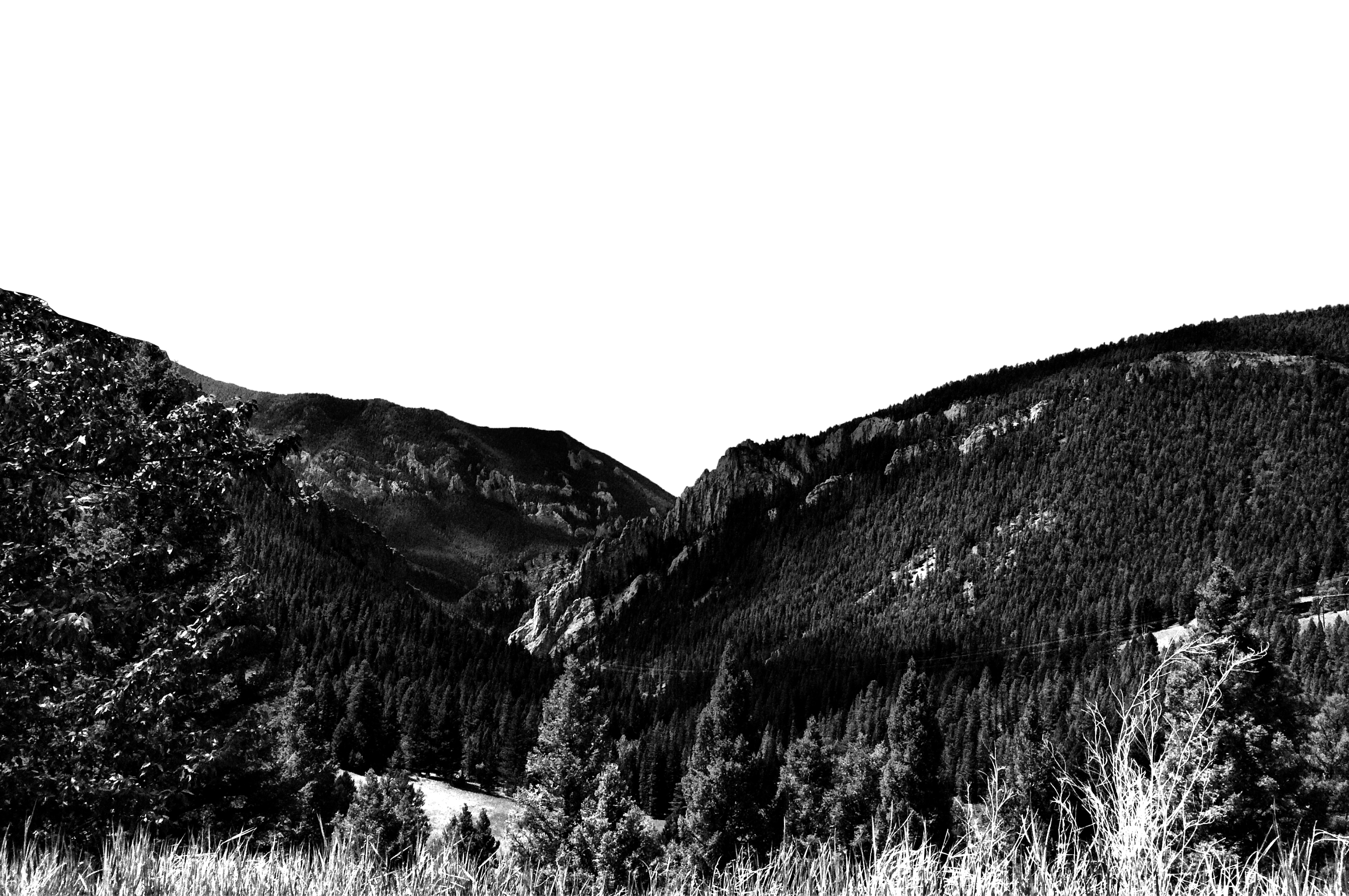This black-and-white photograph features a stark and dramatic landscape with a pure white sky contrasting sharply against the silhouette of a mountainous ridge. The horizon showcases two prominent mountains separated by a descending valley. Both mountains are densely covered with diverse trees, forming an almost continuous forest up to their rugged rock cliff edges. The foreground reveals a field of wild oat, with whitish-gray stalks emerging from the ground. Super tall trees dominate the left side of the image, accompanied by smaller evergreen trees, giving a sense of scale to the scene. The photograph captures a serene yet imposing natural environment, emphasizing the grandeur and scale of the mountains and their forested slopes.